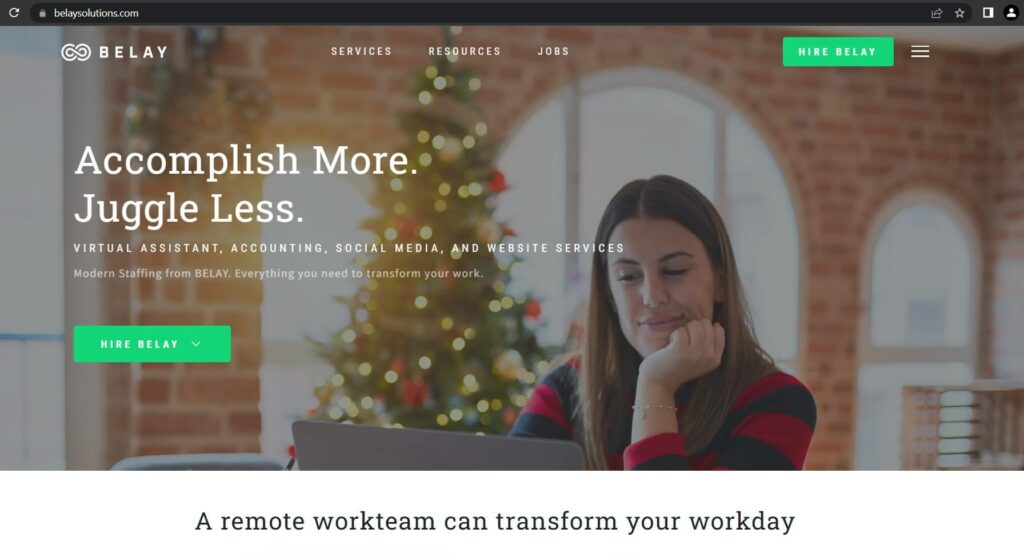The webpage shown in the address bar is BelaySolutions.com. Just below, an infinity symbol shaped as a double infinity signifies the Belay logo, followed by menu options: Services, Resources, and Jobs. A green button, with unreadable text, is seen alongside several bars, possibly representing a menu or navigation option.

The main image features a woman wearing a black and red striped sweater, seated at a desk working on her laptop. She rests her chin on her hand, appearing thoughtful, with a Christmas tree visible behind her in a brick-walled room. Sunlight from outside suggests it’s either sunny or near sunset.

On the left side of the image, text reads: "Accomplish more, juggle less. Virtual assistants, accounting, social media, and website services. Modern staffing from Belay, everything you need to transform your work." Below this, a green button with white, albeit blurry, text possibly says something like "Get Belay" or "Join Belay."

In the top right corner of the webpage, a person icon is displayed, while a refresh symbol adorns the top left corner.